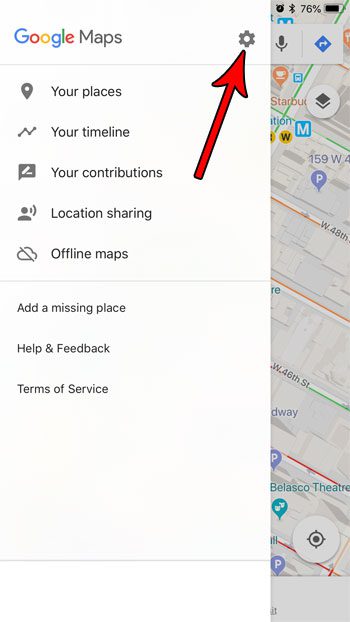The image displays the sidebar of Google Maps on a mobile device. On the right side of the screen, the map itself is visible, showing details such as metro stations and Starbucks locations, indicating a New York City area, specifically around 48th Street and 46th Street. 

On the left portion of the screen, a white sidebar slider is shown. At the top, "Google Maps" is prominently displayed, accompanied by a gear icon to the right, presumably for settings. Below the title, a horizontal line separates it from a list of options accompanied by icons: "Your places," "Your timeline," "Your contributions," "Location sharing," and "Offline maps." Another horizontal bar follows this section.

Further down, additional options are listed: "Add a missing place," "Help and feedback," and "Terms of service," followed by another horizontal gray bar at the bottom. A red arrow outlined in black points to the gear icon at the top, emphasizing its location. Indicators for battery level and Bluetooth are present on the right side, confirming the device is mobile. The map background also shows customizations for map style and location settings.